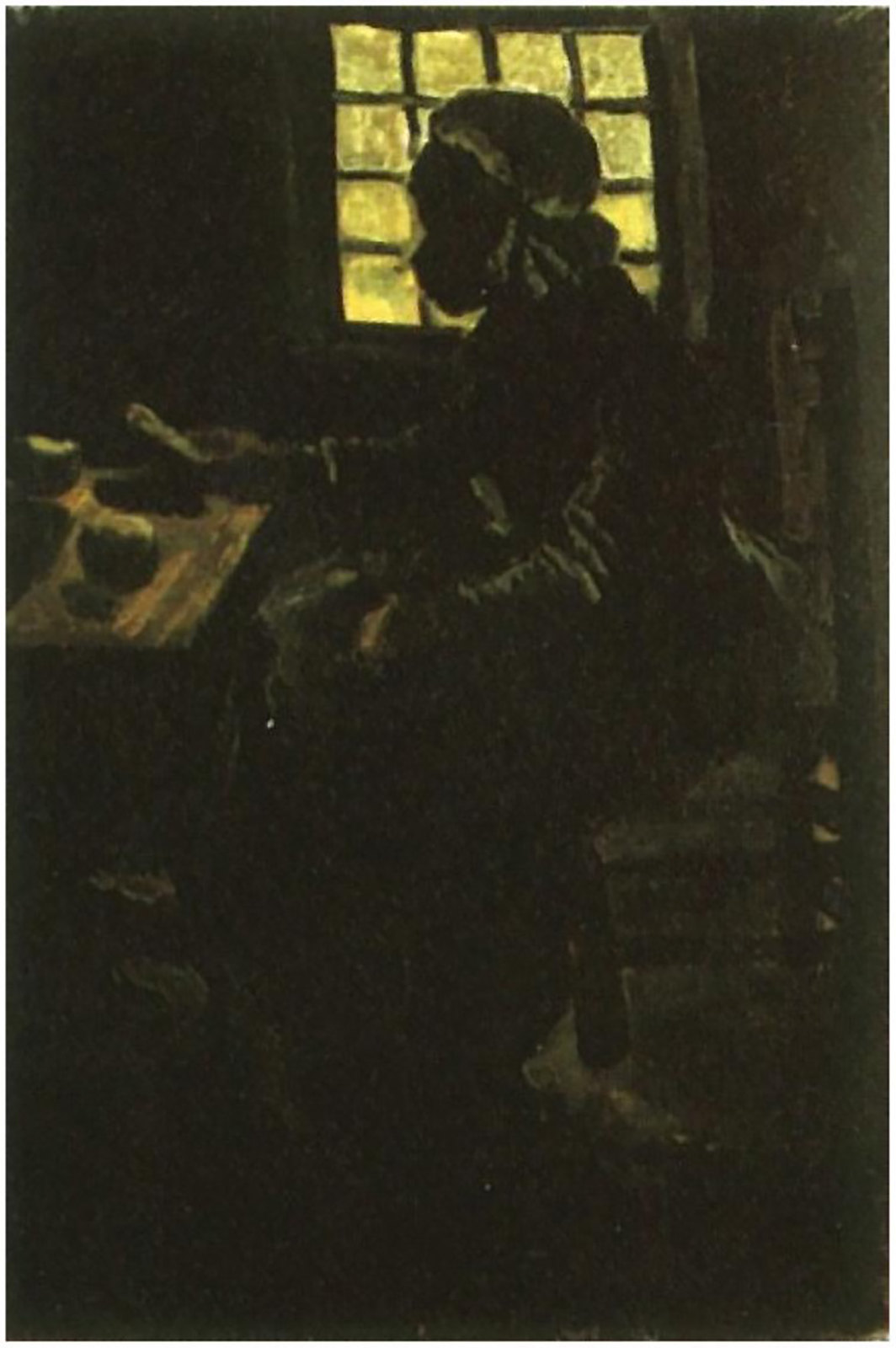In this very dark, shadowy image, reminiscent of colonial times, a woman sits in a dimly lit room, facing left. Her figure is defined mainly by her dark outlines, making her appear almost as a sketch or a painting. She wears a long dress and a bonnet. The scene captures her seated at a wooden table, holding something in her right hand and appearing to examine it. The table presents various indistinguishable objects, with some possibly being food items.

Her chair, with visible wooden legs and back, stands out against the darkness. Behind her, a square window divided into eight panes by wooden frames lets in a faint light, casting a slight yellow tint and creating a stark contrast with the overall dark ambiance of the room. The walls around the window are almost entirely black, contributing further to the eerie, historical feel of the image.